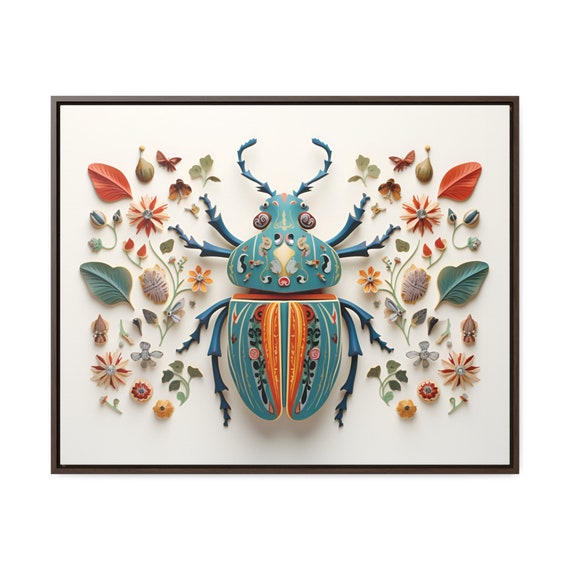The artwork in question is a highly detailed and vibrant painting of an ornate beetle. This centerpiece beetle boasts a stunning blue body adorned with intricate designs in shades of orange, red, green, and yellow, giving it an almost otherworldly charm. The beetle's limbs are depicted in a darker blue, accentuating its detailed structure, while it features prominent white eyes and antennae projecting from its head. Surrounding the beetle are an array of natural elements, including orange and red flowers, green and red leaves, yellow flowers, stems, and butterflies. These elements are carefully placed around the beetle, creating a mirror-image effect from one side to the other. The entire scene is set against a white background and is framed within a thin gray outer frame with a hint of black on the inside. The artwork's presentation in a black wooden frame suggests it could be a digital or three-dimensional piece, giving it a unique and captivating presence as if it were a high-value decor item meant for wall display.